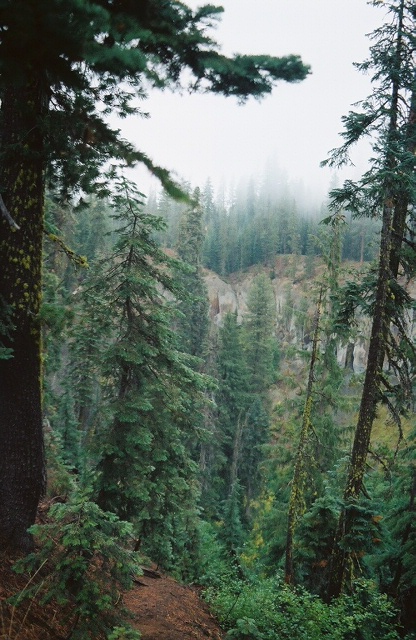This vertical, portrait-oriented photograph captures a scenic, downward view from the top of a hill overlooking a valley characterized by a rugged, hilly, and forested landscape. The foreground features a narrow brown dirt path that traverses the scene, bordered on the left by a substantial pine tree and on the right by a tall, slender tree. This tree exhibits a few sparse, scraggly limbs near its top, adorned with moss or vine. The right side of the path slopes sharply into a deep ravine, contrasting with the pine-studded rocky cliffs opposite. In the background, a misty fog enshrouds the trees atop a sloping rock mountain, adding to the tranquil, high-altitude atmosphere, suggestive of early morning dew or clouds gently cloaking the forested peaks in the distance.